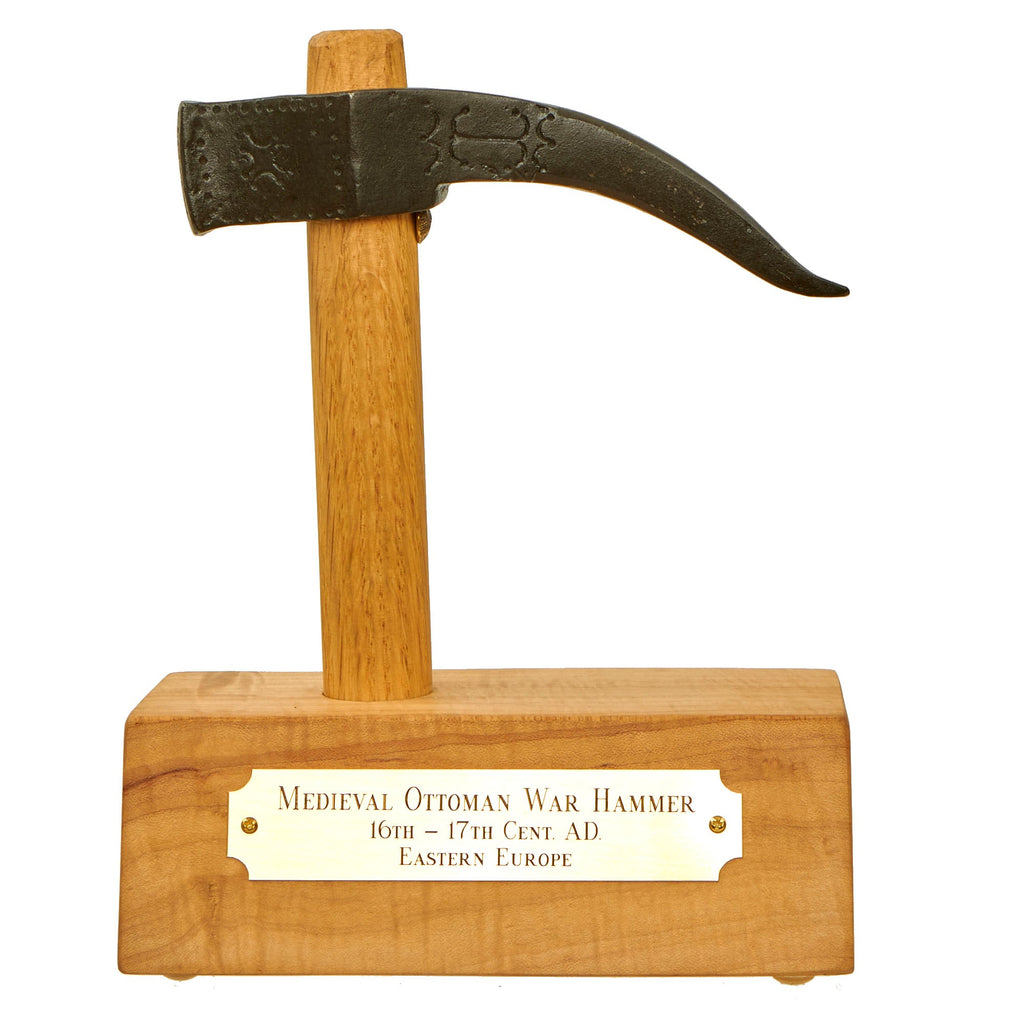The photograph displays a Medieval Ottoman Warhammer from the 16th to 17th century A.D. in Eastern Europe. The warhammer has a distinctive black metal head attached to a light-colored wooden handle. The hammer head is spear-like in shape and appears firmly set into a wooden block base. A golden plaque, made of a light-colored bronze, is affixed to this base, with text in all capital letters and a serif style font, providing details about the artifact. The first letter of the inscription is noticeably larger than the rest. The plaque reads: "Medieval Ottoman Warhammer, 16th to 17th century A.D. Eastern Europe."